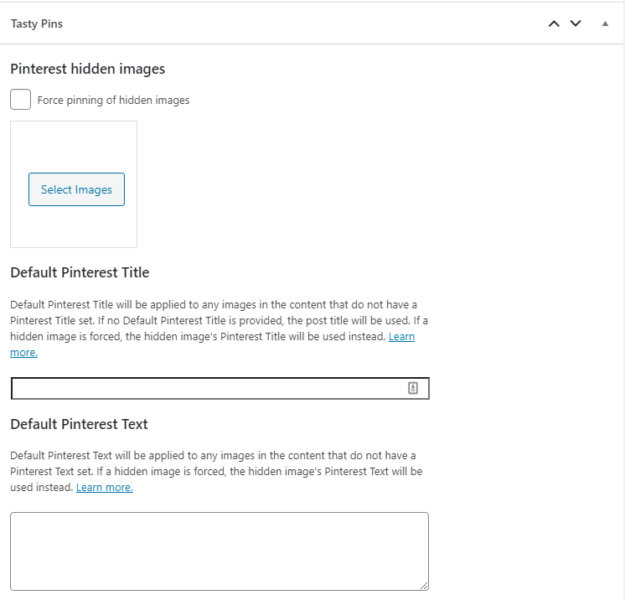The image features a user interface with a clean and structured design presented on a white background with black text. 

In the upper left corner, there is a grey bar stretching horizontally across the width of the screen. This grey bar contains the text "Tasty Pins" in black. On the right side of the bar, there are three arrow icons: an up arrow, a down arrow, and a smaller up arrow. 

Below this bar, there is another thin grey line spanning from left to right. Underneath this line, "Pinterest Hidden Items" is written in bold black text. 

Directly below this, there is an empty grey box. Accompanying the box is grey text that reads "Forced pinning of hidden images."

Further down, there is another grey box, which includes a blue box inside it. The blue box contains the text "Select Images" in blue font.

Under this box, the text reads "Default Pinterest Title," followed by a description: 
"Default Pinterest title will be applied to any images on the content that do not have a Pinterest title set. If no Pinterest title is provided, the post title will be used. If a hidden image is forced, the hidden image's Pinterest title will be used." 

Immediately following this description, there is an underlined blue text link labeled "More Info."

Farther down the interface, there is a black-outlined search box currently empty. Below this box is another section titled "Default Pinterest Text," followed by a corresponding description: 
"Default Pinterest text will be applied to any images of content that do not have a Pinterest text set. If a hidden image is forced, the hidden image's Pinterest text will be used instead." 

There is another underlined blue text link labeled "Learn More." 

At the very bottom, there is a light grey-outlined area intended for text input, which is currently empty.